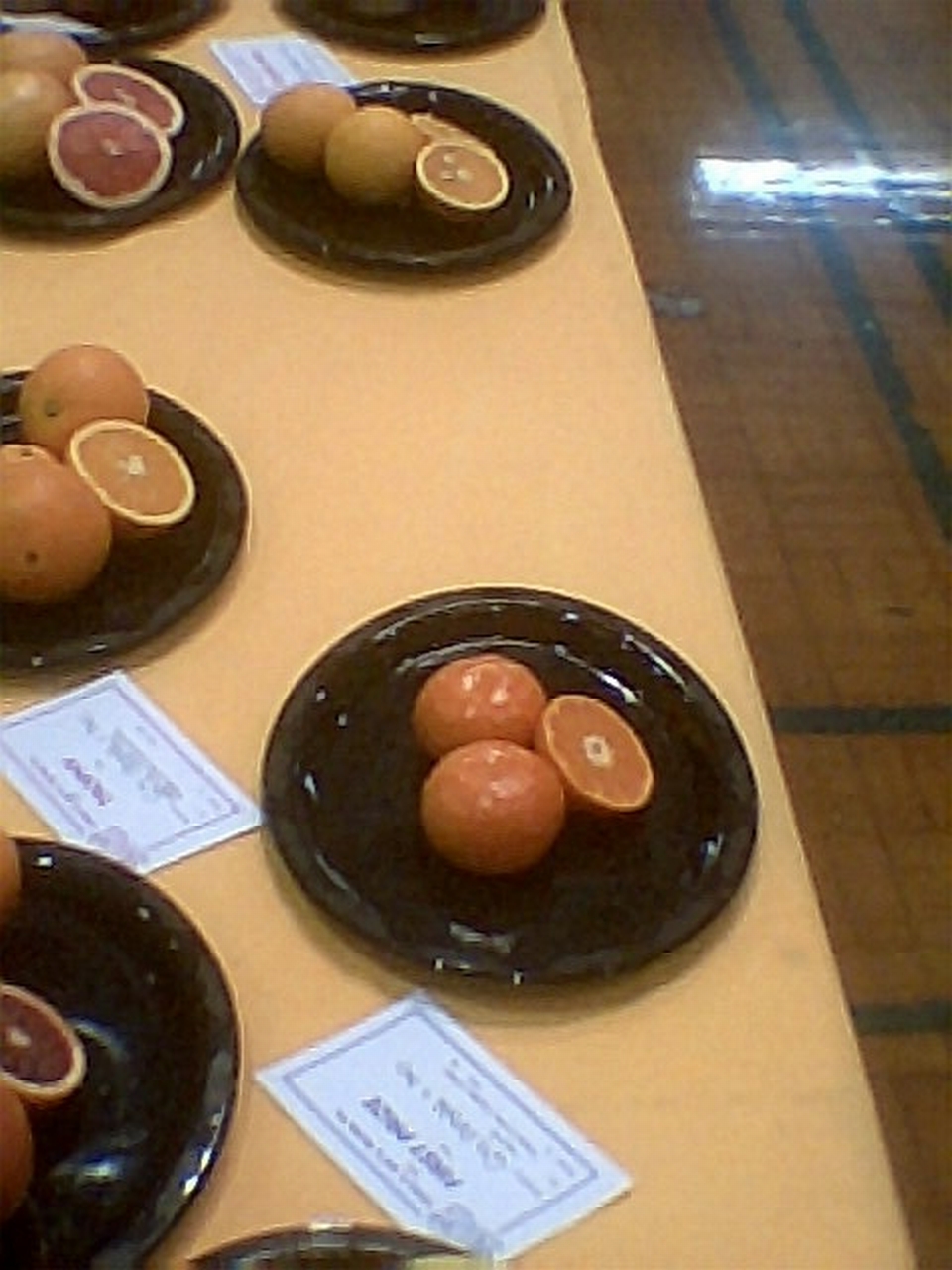The image is a detailed color photo featuring five black plates arranged on a long, orangish-tan table. Each plate holds citrus fruits, including oranges and grapefruits, with several fruits displayed whole and others cut in half to reveal their vibrant interiors. Notably, the top left corner showcases sliced grapefruits, while the plates on the right display sliced oranges. Visible next to each plate are white, postcard-sized labels with bordered edges, likely indicating the names of contestants and fruit varieties. The setting appears to be a county or state fair, suggested by the polished wooden floor and diploma-like labels, highlighting a contest or display of citrus fruits.